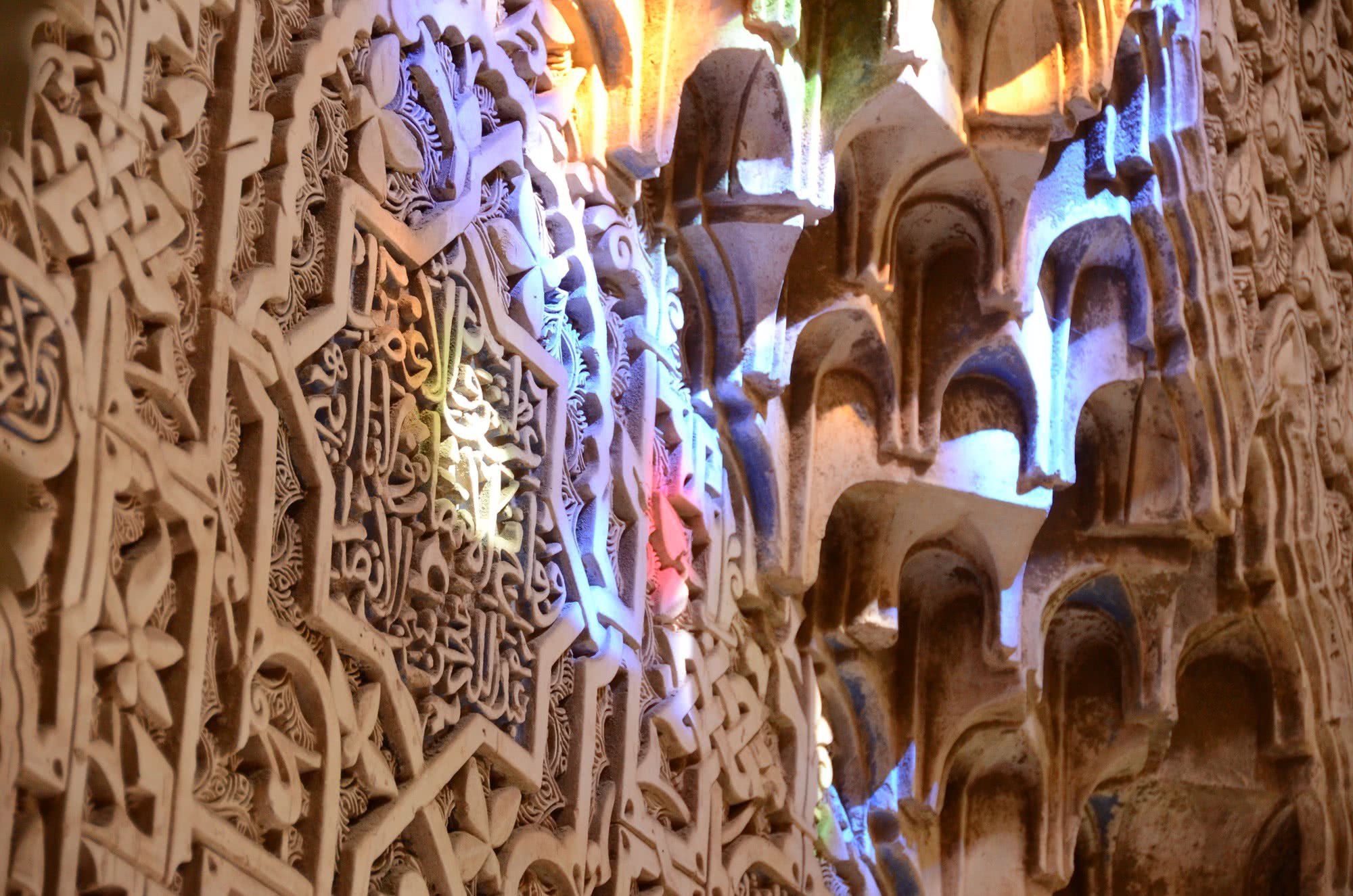The image depicts an intricately designed sand-colored wall, possibly part of a Hindu temple, adorned with elaborate clay formations and human-like sculptures wearing headdresses. Dominating the right side is what appears to be a delicately crafted construction featuring these figures. On the left, there is a prominent engraving that resembles a Star of David, surrounded by intricate writings that might be in Arabic. The setting is bathed in a myriad of colors, including shades of red, purplish-blue, purple, blue, orange, yellow, green, and sandy gray. Toward the top middle, vibrant purple and blue lights, along with bright pink hues, cast an otherworldly glow on the wall, enhancing the overall mystical ambiance of the scene.